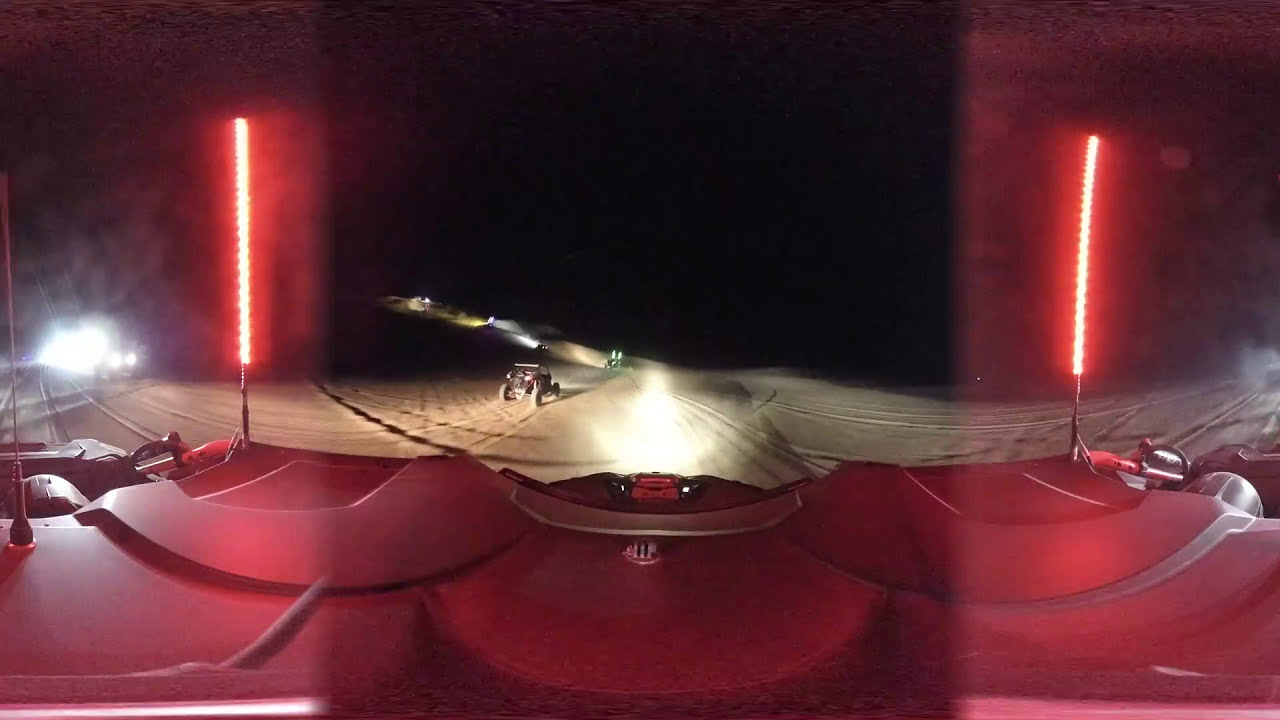This is a wide-angle panoramic photograph taken at night from the viewpoint of a vehicle's dashboard. The foreground of the image features the dash of the car, with a pair of red lights on either side that illuminate with yellow borders. The car's headlights cast their beams down a road or a sandy terrain, with noticeable snow and tire tracks suggesting either a road or a wintery landscape. To the left of the left red light, there are headlights from another vehicle, indicating the presence of multiple vehicles. Ahead of the primary vehicle, there is another car or dune buggy, part of a line ascending a sand dune or snow-covered hill. Bright lights highlight these distant vehicles, making them visible against the pitch-black nighttime sky. While the exact type of green object from which the image was taken is unclear, it could be an off-road buggy given the context of other vehicles and the scene. The scene suggests a dramatic, possibly competitive night rally or dune buggy race with an array of illuminated vehicles driving uphill into the darkness.